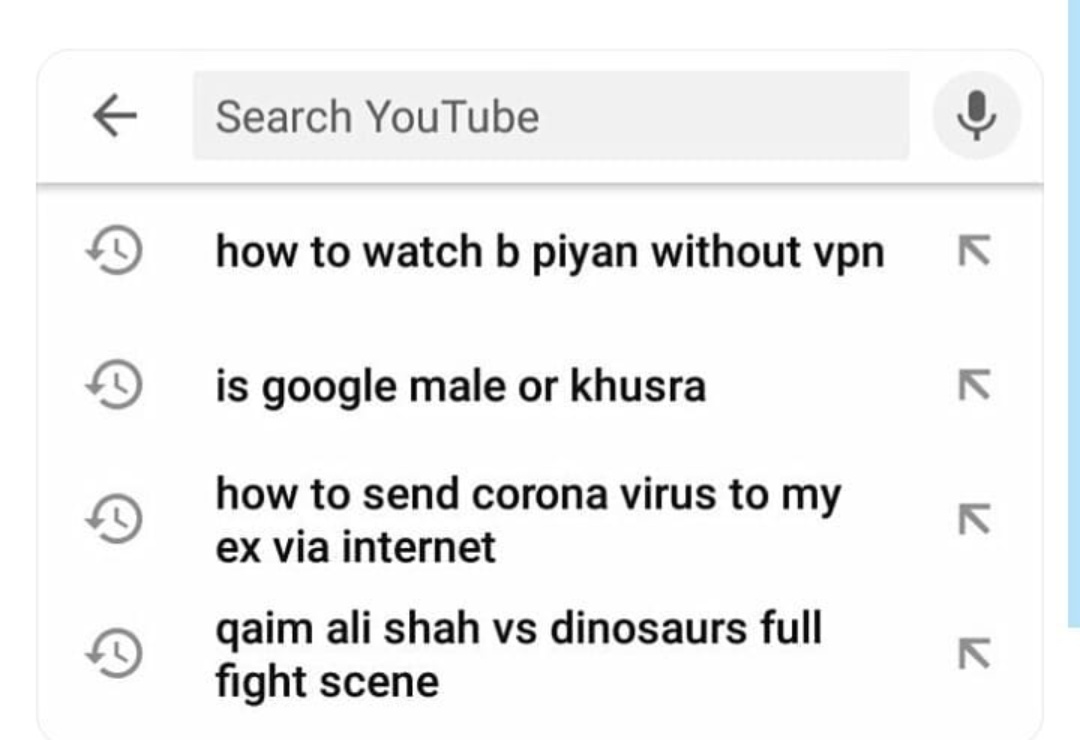This detailed image captures a screenshot set against a minimalist white backdrop. At the top, a white bar prominently displays a search bar in light gray, with the placeholder text "search YouTube" in a subtle gray font. To the right of this search bar, a sleek microphone icon is encased within a light gray circle. On the left side of the search bar, an arrow icon points left, hinting at navigation functionality. 

Directly beneath this bar, a thin, light green line underscores the top section, leading into a list of search queries displayed in bold black text. The first query reads, "How to watch Bee Pien without VPN," providing a clear and straightforward question. Following this, the phrase "Google Mail or Kusra" is listed. Subtly shocking, the next query states, "How to send coronavirus to my ex via internet." Finally, a more whimsical search is shown: "Qaim Ali Shah vs dinosaurs full flight scene."

A light blue borderline lines the right side of the screenshot, extending vertically from the top to the bottom, framing the image with a subtle touch of color.